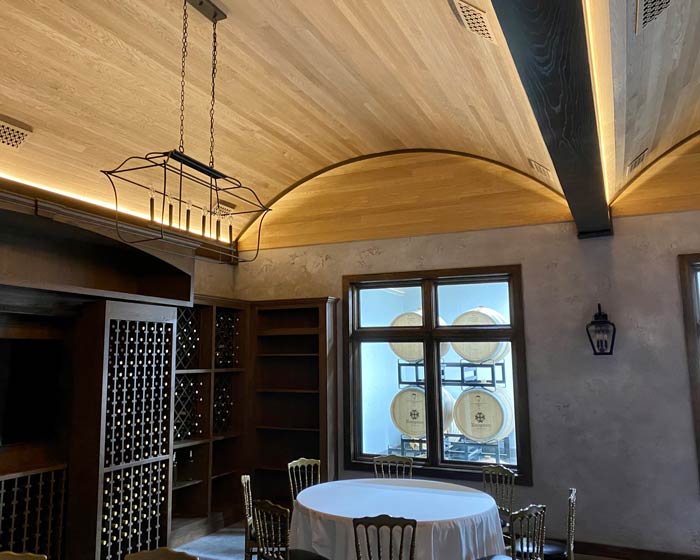The photograph captures the elegant interior of what appears to be a wine-centric restaurant or perhaps a sophisticated storage space. On the left wall, there is an expansive wooden cabinet boasting numerous small, individual compartments, meticulously filled with wine bottles. This cabinet includes both vertical and crisscross shelving to accommodate the bottles, showcasing them in an organized and visually appealing manner. 

The room is adorned with beautiful mahogany furniture and shelving, contributing to the warm and inviting atmosphere. The ceiling is a notable feature, composed of light-colored wooden slats arranged in a concave, sine wave pattern, with recessed lighting elegantly integrated along the center beam. 

A round table covered with a white tablecloth is positioned with seven wooden chairs around it, indicating a dining or tasting area. A modern, industrial-style chandelier with black elements hangs above, enhancing the refined ambiance. Additionally, a classy black lantern is mounted on the wall, though it is currently unlit.

The back wall is white, and it features dark wood-framed windows that offer a view into another space. This adjacent area displays the ends of oak wine barrels, which appear new and are supported by wooden structures. Sunlight from the blue skies filters through, hinting at an outdoor setting or a cleverly designed adjoining room, reinforcing the central theme of wine. The scene exudes sophistication, with wine clearly playing a significant role in the room's purpose and design.